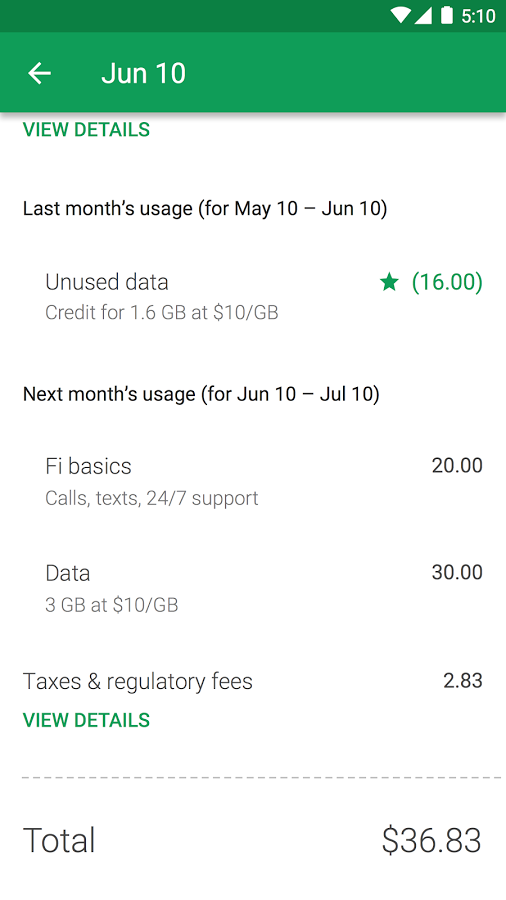A mobile device screen showcases various details regarding Wi-Fi signals, battery status, and data usage. In the top-left corner, there is a Wi-Fi symbol, while the battery icon shows a 510 value next to the left arrow. The date displayed is June 10th. 

A green rectangle labeled "View Details" is present, accompanied by black text stating "Last month's usage for May 10th to June 10th." Below this, grey text indicates "Unused data credit for 1.6 gigabytes at $10 per gigabyte."

Underneath, an asterisk followed by the number 16 in parentheses appears. Further black text reads "Next month's usage for June 10th to July 10th."

The following section outlines "Wi-Fi basics, calls, text, 24-7 support" with a price of $20 marked in black, followed by a separate text indicating "Data: 3 gigabytes at $10 per gigabyte, $30." The regulatory fee of $2.83 is also noted.

A green "View Details" button is included, along with a section of dash marks leading to a "Total" button. The total amount is specified as $36.83 on a white background. The date June 10th is reiterated at the end.